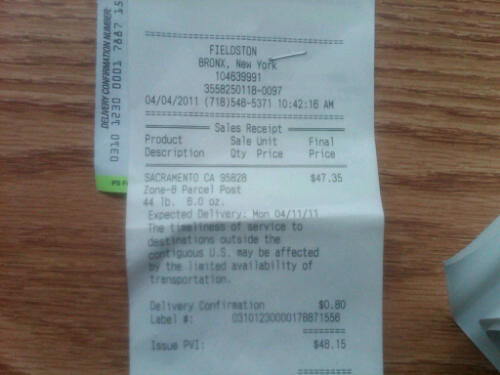On a light wooden table, there lies a white receipt with crisp black typography. The receipt, prominently featuring the name "Fields-Ton Fieldston" in Bronx, New York, is stapled in the middle to an unseen secondary paper, suggesting it might be a multiple-page document. The receipt is dated April 4, 2011, and lists various transaction details, including the store and time stamp. It appears to be a comprehensive sales report detailing product descriptions, sales units, final price, and a location identifier as Sacramento, CA with the zip code 4735. Further down, there are logistics notes indicating an expected delivery date of April 11, 2011, along with a delivery confirmation, label number, and an issued PVI, ensuring all information for the transaction and consequent shipment is meticulously documented.